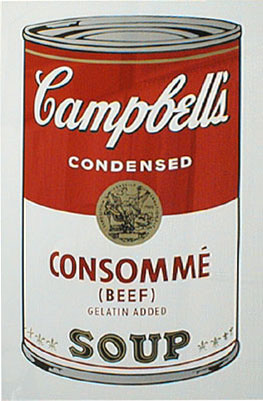This artwork features a detailed artist’s rendition of a Campbell’s soup can, set against a light gray or white background with a design that suggests it might be a drawing or painting. The can's proportions are approximately twice as tall as it is wide. At the top, the can features Campbell’s signature cursive logo in white within the red upper half, with the word "condensed" in the same white font underneath. Separating the red upper half from the off-white lower half is a golden seal, which seems to depict an image, possibly a female figure. The lower half of the can contains the word "consommé" in red letters with a small accent over the "e", followed by "beef" and "gelatin added" in parentheses. At the very bottom, the word "soup" is displayed in black letters outlined with a gold trim. To the sides of the word "soup", there are four gold stars on each side. The bottom rim of the can appears to be gray.